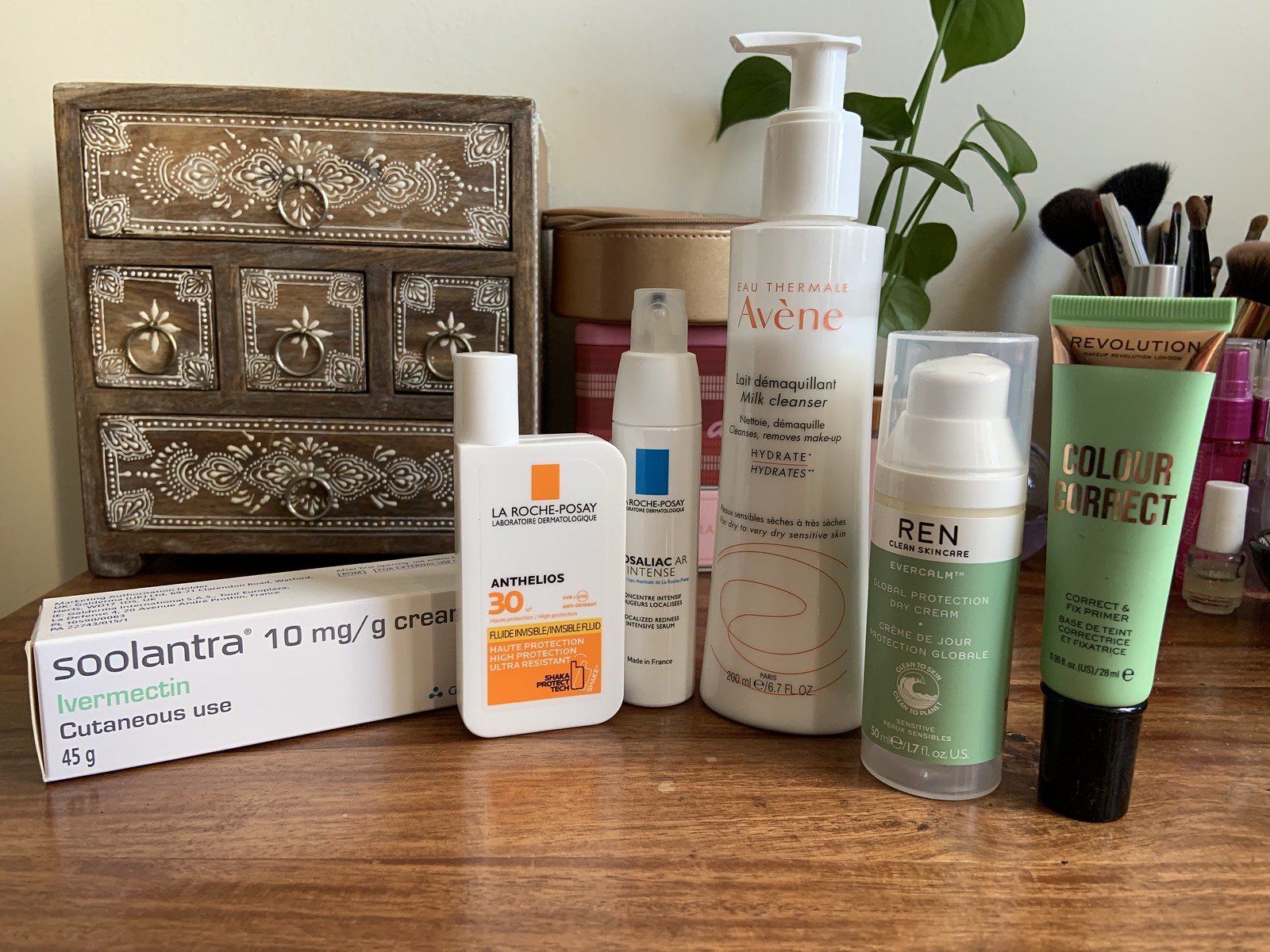The image depicts the interior of a house, focusing on a section of a medium brown wooden table with a prominent wood grain design, set against a stark white wall. The table holds a variety of objects, each meticulously detailed. 

On the left side of the table sits an antique-looking jewelry box, crafted from brown wood and adorned with ornate white detailing. The jewelry box features five drawers, each with a small, round silver pull tab, adding a touch of elegance to the vintage piece.

To the right of the jewelry box is a white box labeled "Soolantra 10 mg/g Cream," an ivermectin medication weighing 45 grams. Positioned next to the Soolantra box is an assortment of skincare products, including a cream by La Roche-Posay. Alongside it is a longer tube labeled "Milk Cleanser," followed by a product from REN Clean Skincare named "Evercalm Global Protection Day Cream." Completing the skincare collection is another item titled "Correct and Fix Primer."

In addition to these, there's a small, cylindrical jar containing various makeup brushes, indicating the presence of a personal grooming routine. The detailed arrangement of these items provides a glimpse into the homeowner's daily regimen and aesthetic preferences.